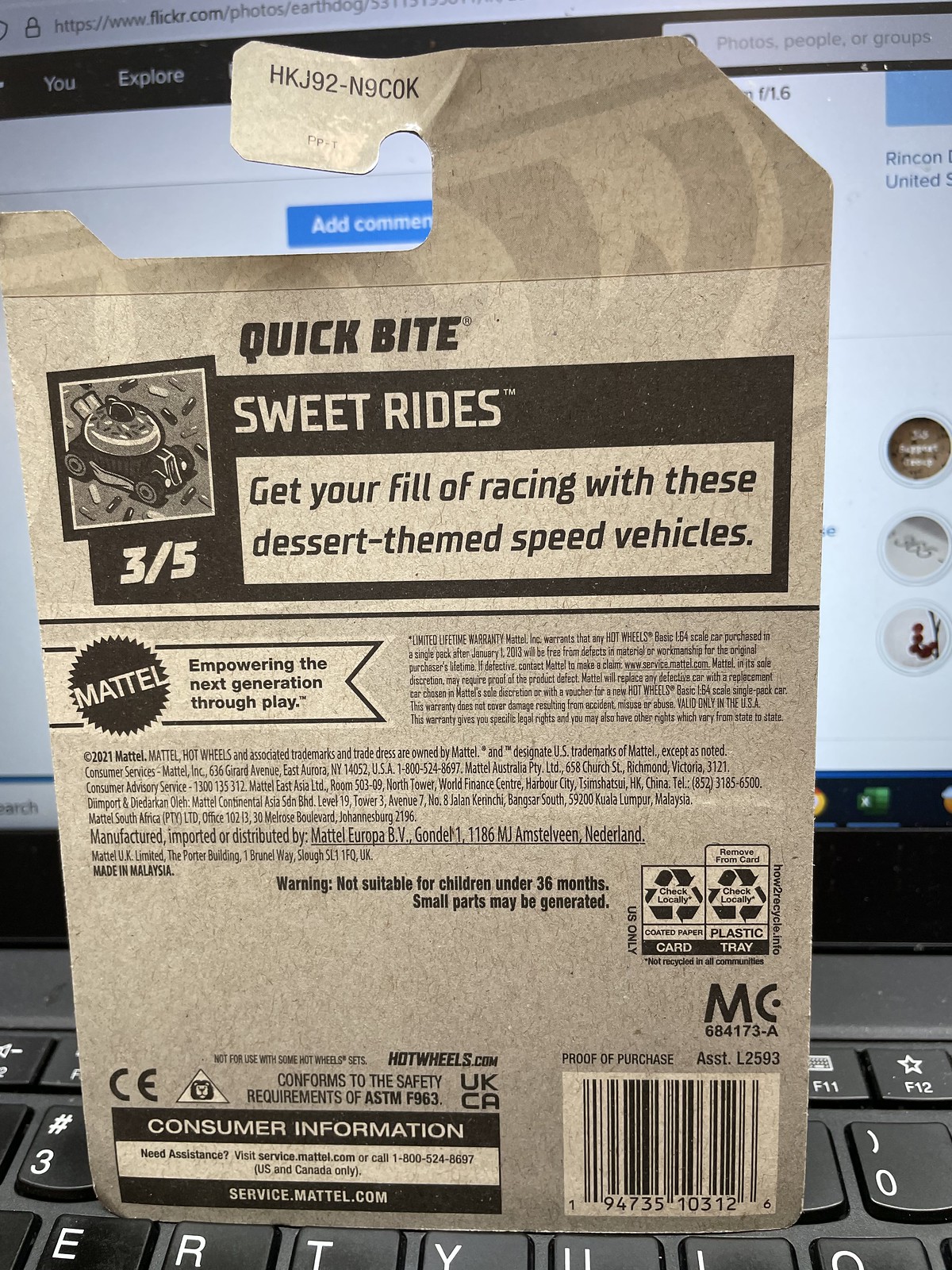The image depicts a cardboard-backed product positioned atop a laptop. Visible details of the laptop include the keyboard spanning from the 'E' and 'R' keys to 'I' and 'O', including the number keys and function keys up to F12, while the screen partially displays a webpage, likely Flickr.com, blocked by the cardboard product. 

The product is a Mattel toy car package, which features prominently on the brown cardboard the text "Quick Byte" and below it, "Sweet Rides: Get your fill of racing with these dessert-themed speed vehicles." There is an illustration of one dessert-themed car, labeled "3/5", and to the right, there is the Mattel logo with the tagline "Empowering the next generation through play." 

Additional details on the packaging include fine print with legal and consumer information, recycling symbols, a barcode, "proof of purchase" text, and various warning labels like "Not suitable for children under 36 months" and safety conformity notes such as ASTM F963. The barcode reads "194735103126", and there are codes and warnings indicating recycling instructions. It is also marked with "Hot Wheels" branding and the CE logo, with disclaimers about compatibility with certain sets. Consumer assistance information is given with a website (service.mattel.com) and a toll-free number (1-800-524-8697).